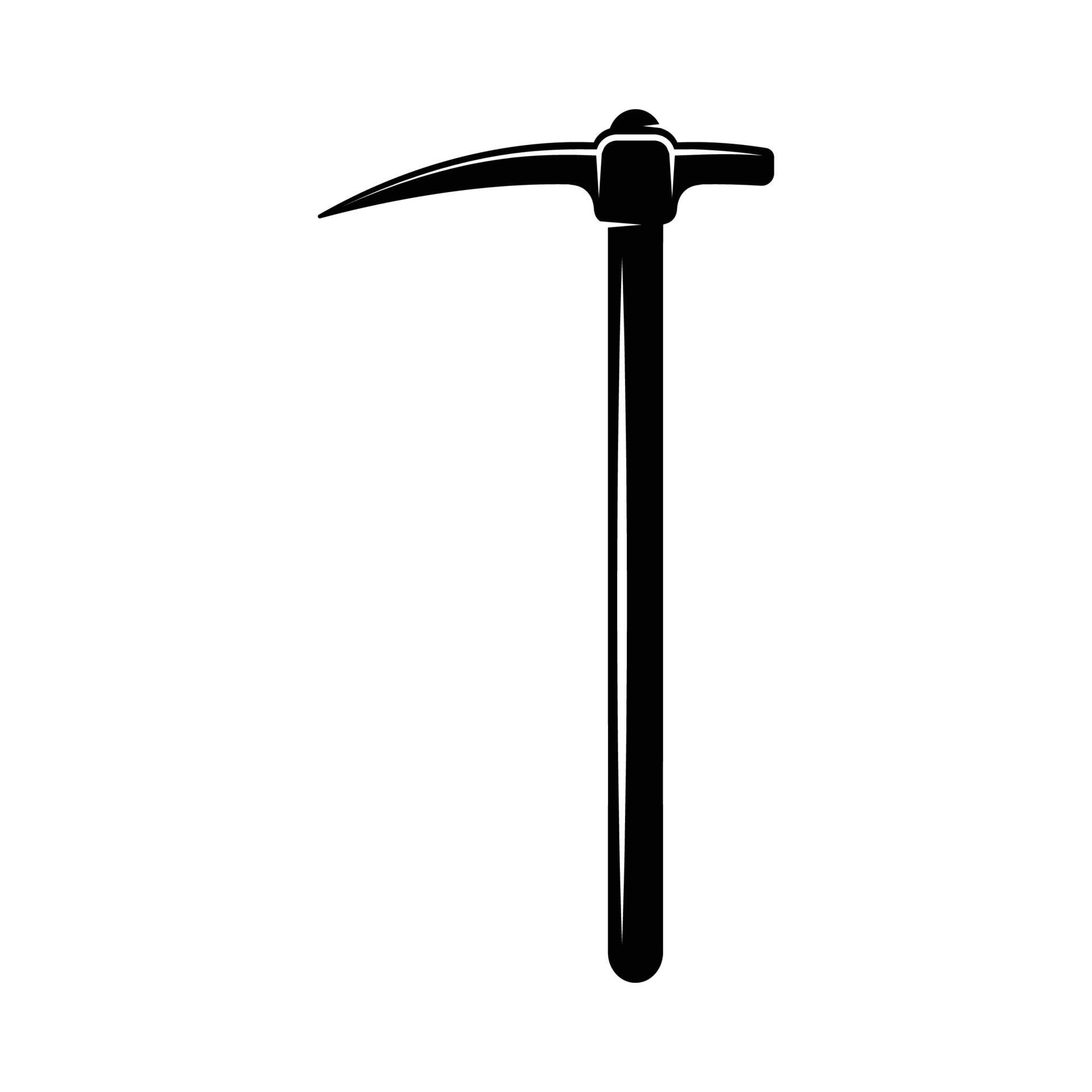The image is a detailed, computer-generated drawing of a traditional pickaxe rendered in solid black with distinct white highlights. The pickaxe stands vertically on a plain white background, dominating most of the space. It features a long, slender handle with white highlights on the left side and top, suggesting a light source from the left. The pickaxe head is divided into two ends: the left side is sharp and pointed, while the right side is blunt and squared, with slightly rounded edges. The overall design is reminiscent of a vector graphic, emphasizing its clean, minimalistic, and monochromatic style.